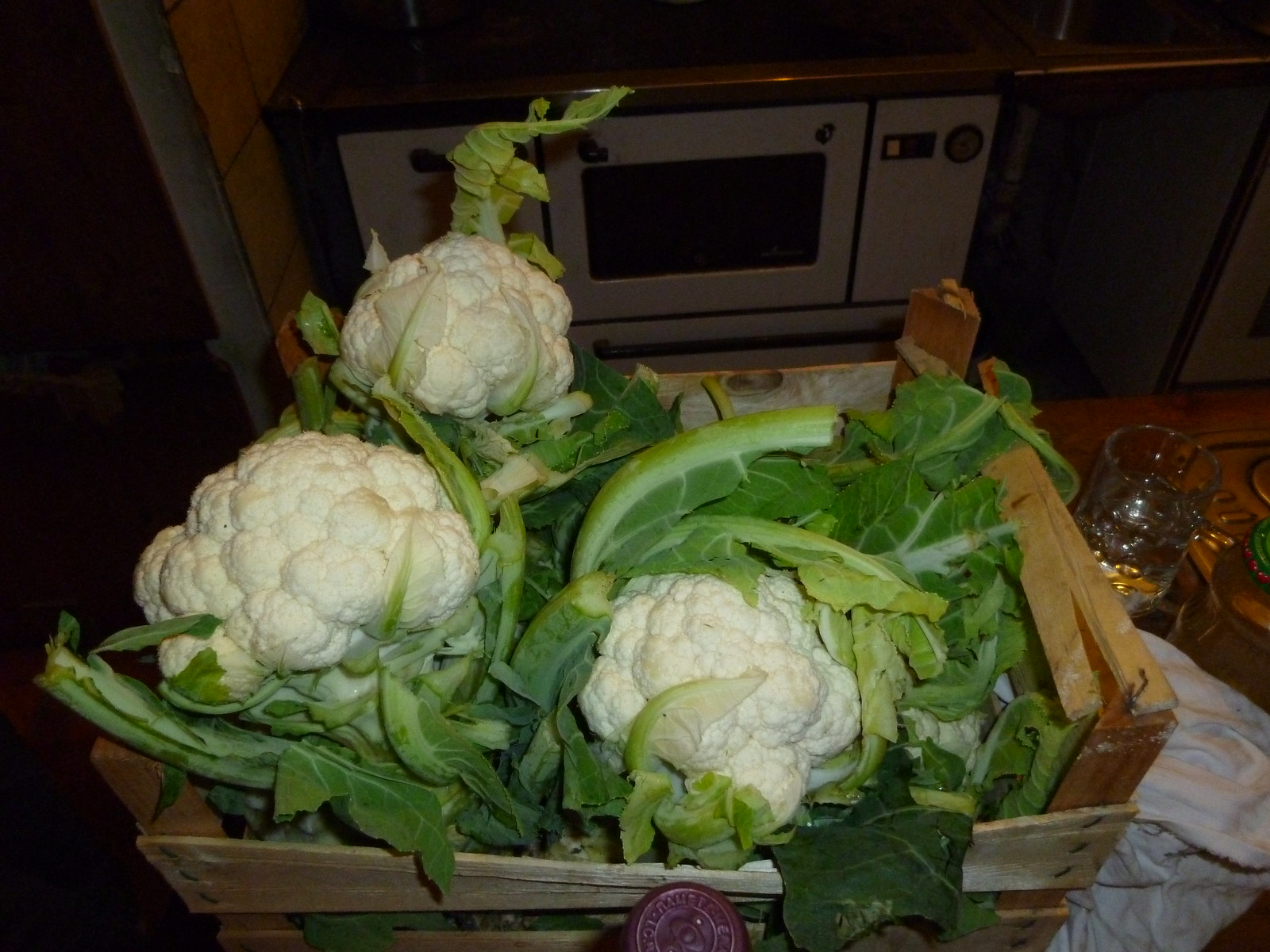The photograph, taken inside a dimly lit kitchen, depicts a rustic scene centered around a wooden basket filled with three freshly picked heads of cauliflower. The vibrant, leafy greens and white heads of cauliflower indicate they are likely organic, recently bought or harvested. The cauliflowers rest on a white cotton towel placed underneath the basket, which also sits on a dark brown counter. To the left of the basket stands an empty, clear glass, and a purple-topped soda bottle is visible just below the basket. The kitchen background features appliances such as an oven and possibly a microwave or toaster oven, adding to the cozy, homely atmosphere. The flooring is wooden, and the edge of a doorway is faintly visible, hinting at other parts of the home.